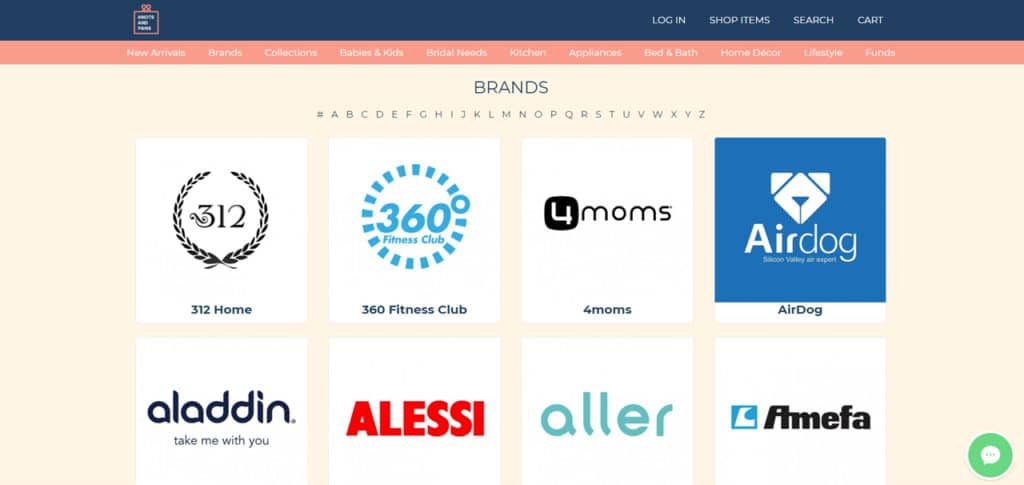The image showcases a well-organized e-commerce webpage, featuring a variety of clickable links and categories designed to enhance user navigation. Key categories are prominently displayed, including "New Arrivals," "Brands," "Collections," "Babies and Kids," "Kitchen," "Appliances," "Bed and Bath," "Home Decor," "Lifestyle," and "Phones." 

The top-right corner of the page includes essential user options such as "Login," "Shop Items," "Search," and "Cart," providing easy access to user account management and shopping functionalities.

Several reputable brands are highlighted on the page, such as "312 Home," "360 Fitness Club," "4Moms," "A Dog," "Aladdin®," "Take Me With You," "Alessi," "Alaa," and "Amifar," signifying a diverse product range available for online shoppers.

Overall, the webpage design appears to be intuitive and user-friendly, aimed at catering to a wide array of consumer needs and preferences.